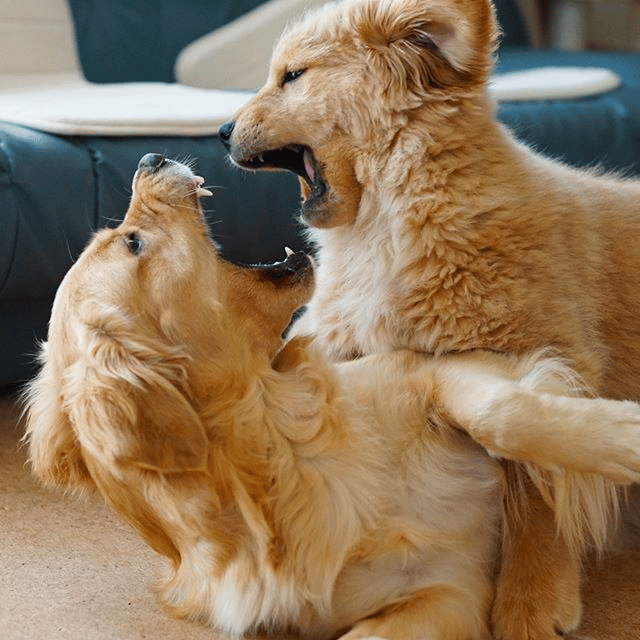This photograph captures a playful scene between two golden retrievers inside a house. The larger dog, presumably an adult, is laying on a beige carpet with its head facing straight up and its mouth wide open, revealing all its teeth in what appears to be a playful snarl. The smaller, younger golden retriever, with its ear adorably flipped from their playful tussle, is positioned on top of the larger dog, also with its mouth wide open. Both dogs, sharing a beautiful honey-colored coat, are staring directly at each other, clearly enjoying a spirited play fight. They are lying in front of a piece of dark furniture or possibly a green leather sofa, providing a cozy indoor backdrop to their exuberant interaction.